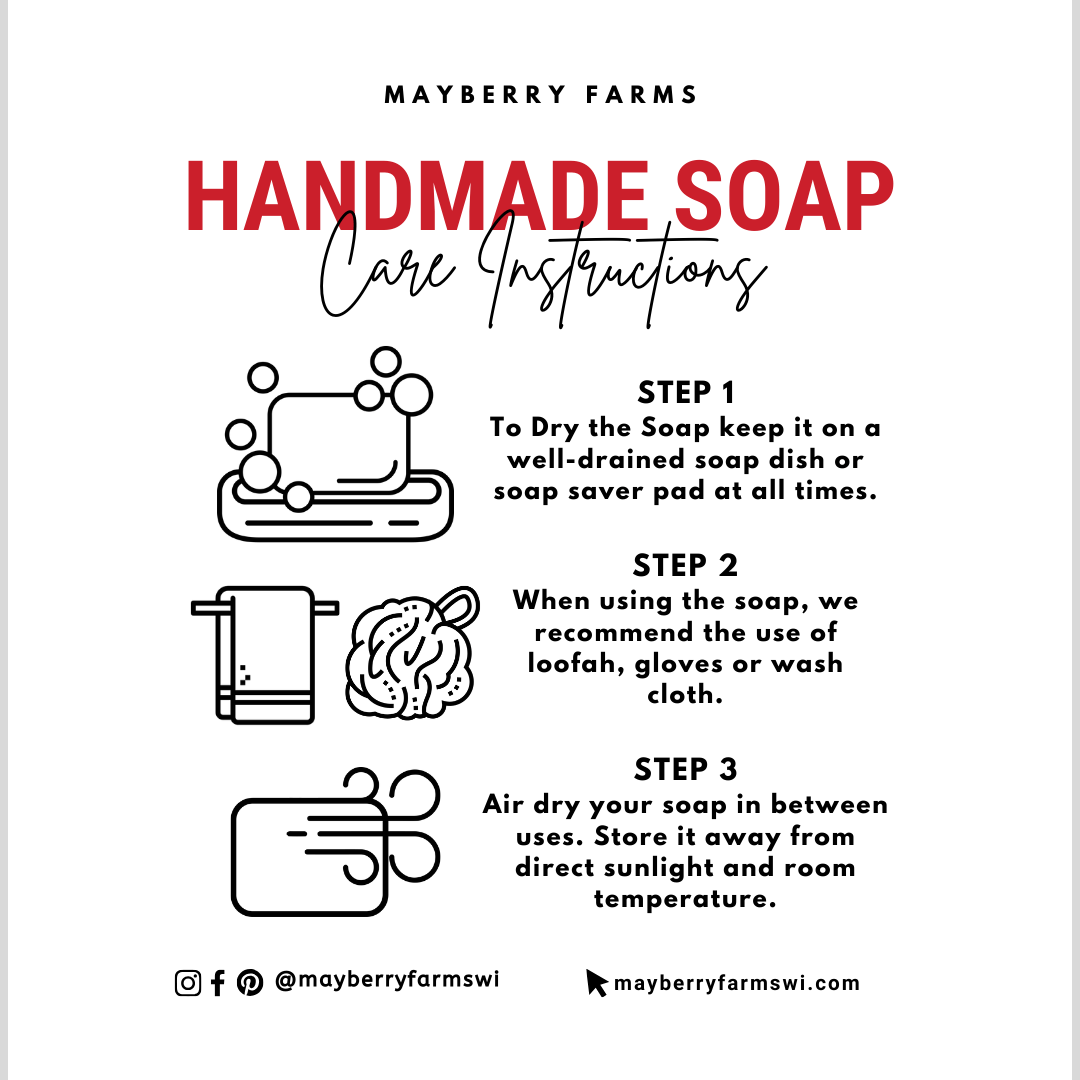This infographic from Mayberry Farms provides detailed care instructions for their handmade soap against a solid white background. At the top in small black text, it reads "Mayberry Farms," followed by "Handmade Soap" in large, bold red font. Below that, in a handwritten style, it says "Care Instructions."

The infographic is divided into three sections, each with respective clip art and instructions:

1. **Step One**: A black line-art image of a soap bar with bubbles in a soap dish. The accompanying text advises to keep the soap on a well-drained soap dish or soap saver pad at all times to dry it properly.
  
2. **Step Two**: A towel hanging on a pole and a loofah. The instructions recommend using a loofah, gloves, or a washcloth when using the soap.

3. **Step Three**: A rectangle with motion lines illustrating the drying process. The text instructs to air dry the soap between uses and store it away from direct sunlight and at room temperature.

At the bottom, social media icons for Instagram, Facebook, and Pinterest are shown with the handle @MayberryFarmsSWL. Additionally, there's an image of a mouse cursor with the website MayberryFarmsSWI.com.